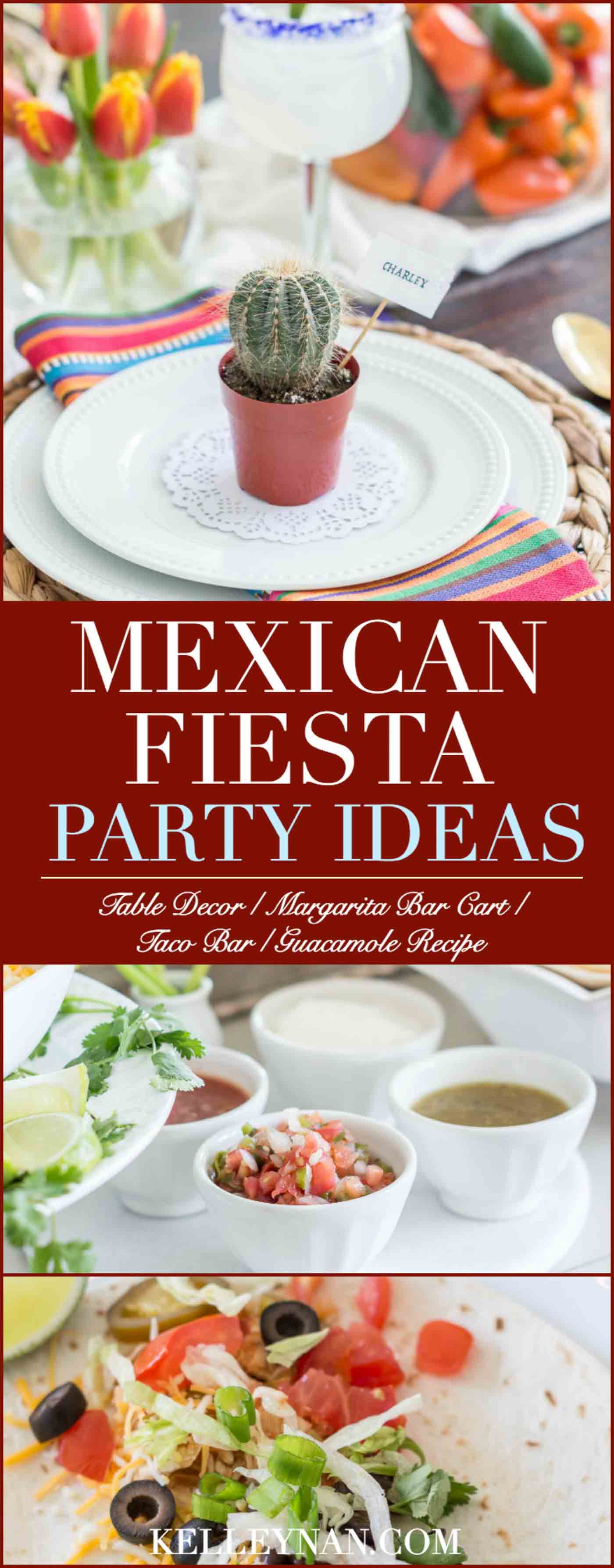This digital poster, reminiscent of a narrow, tall book cover, features vibrant Mexican Fiesta party ideas. The poster is bordered in red and primarily has a series of three photographs that highlight various elements of a festive table setting. 

At the top, a large horizontal rectangular frame displays a detailed table arrangement: a round white plate holds a small potted cactus, surrounded by a margarita glass, flowers, and assorted food items including salad, fruits, and snacks, adding bursts of color and texture to the scene.

Below this image, set against a red background with decorative elements, is key informational text in uppercase and cursive fonts that reads "Mexican Fiesta Party Ideas: Table Decor / Margarita Bar Cart / Taco Bar / Guacamole Recipe," giving a glimpse into the festive theme and culinary inspiration.

The middle section features a photograph of a white plate with four white bowls, each holding different food items, some of which are liquid, further enhancing the culinary diversity featured in the poster.

At the bottom, another photograph showcases chopped vegetables, including onions and tomatoes, meticulously arranged on a surface, hinting at fresh ingredients ready for a fiesta.

Lastly, at the bottom center, in bold white text, the website name "KELINAN.COM" is displayed, making this digital poster not only visually appealing but also informative and a gateway to more fiesta ideas and recipes.